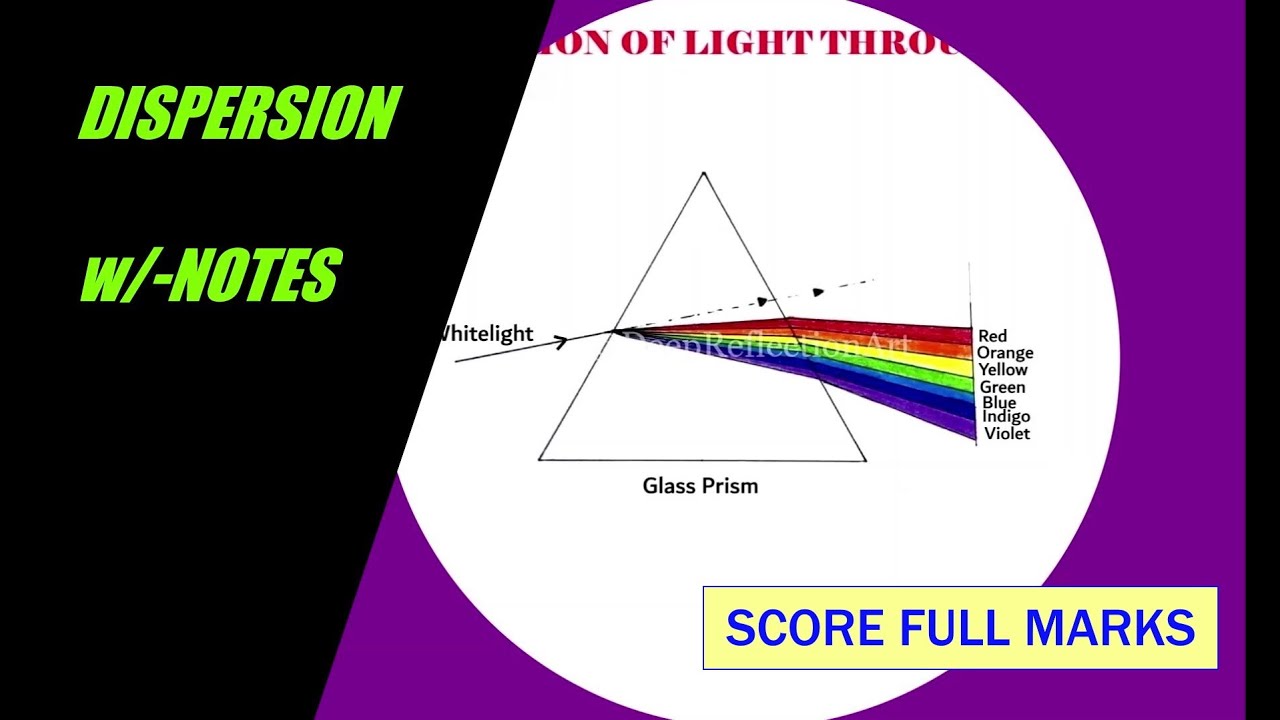The image is a detailed color illustration resembling a slide from a PowerPoint presentation, set against a dark purple background. On the left side of the slide, there is a black trapezoidal section with neon green all-caps text in a sans serif, italicized font, reading "DISPERSION W/NOTES". In the center of the slide, a white circle encompasses a white triangle with a black border, representing a glass prism. At the top of the circle, partially obscured, is the red text "OF LIGHT THROW," with the following words unreadable. An arrow labeled "WHITE LIGHT" points into the left side of the prism. Emerging from the right side of the prism is a detailed rainbow with labels for each color: "RED," "ORANGE," "YELLOW," "GREEN," "BLUE," "INDIGO," and "VIOLET." Below the prism, in black text, it reads "GLASS PRISM." On the lower right side of the slide, there is a yellow rectangular box with a blue border and blue all-caps text stating "SCORE FULL MARKS." The layout is a clear and colorful infographic likely intended for educational purposes.